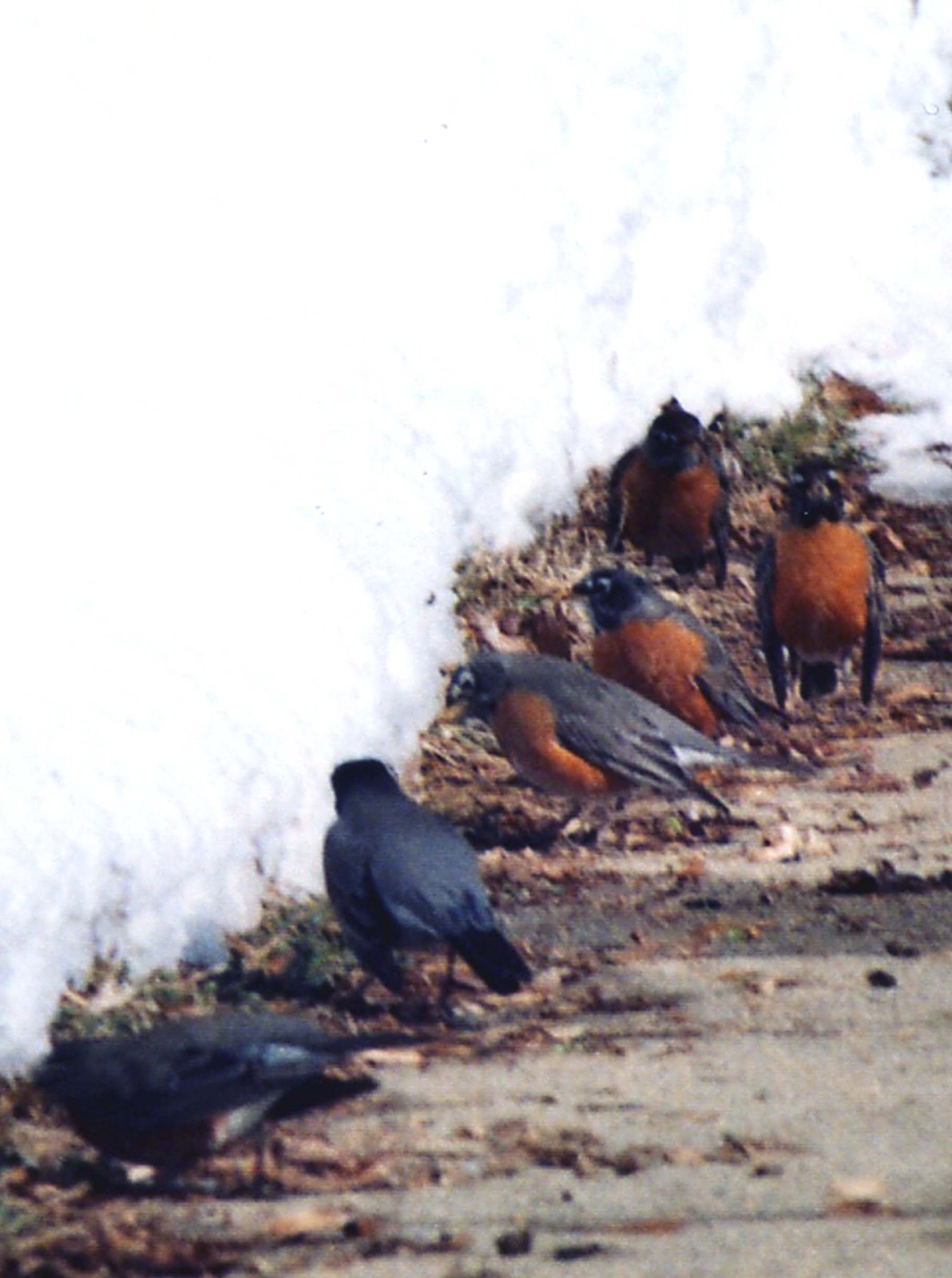The photograph depicts six birds with black wings and backs, and reddish-orange underbellies, believed to be robins. They are standing on a concrete pathway scattered with brown leaves, while the background features a thick layer of snow on the left side, creating a stark contrast against the snow-free ground they occupy. Two of the birds are turned away, showing their backs, while the other four display their vibrant underbellies, with one facing the camera directly. The scene suggests the birds are foraging for food, likely nuts, amidst the stark, snowy landscape.